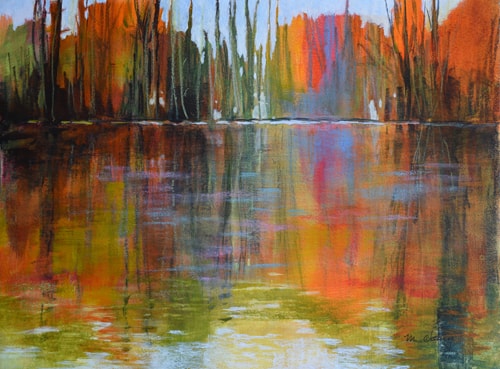This painting, likely a watercolor, is rectangular in shape and features a serene outdoor setting dominated by a pond. At the bottom part of the painting, a murky water body mirrors the vibrant foliage and the sky above, producing a blended palette of greens, oranges, reds, blues, and yellows in the water's surface. The pond's surface, though hinting at a green hue, mainly reflects the diverse colors of the surrounding tree line and shrubs.

Just above the pond, a cluster of plants and trees exhibits a spectrum of colors—green, orange, red, and blue—conjured by broad strokes typical of watercolor art. Individual leaves aren't distinctly visible, replaced instead by amorphous patches of color. The tall stalks and more bush-like formations meld into a harmonious scene. 

The upper section of the painting displays a blue sky visible through the tree canopy. On the painting's left side, the trees show a mix of green and orange hues, with brown and black trunks exhibiting specks of green. The trees and plants in the central and right sections echo this color theme while also incorporating touches of blue. The artist has subtly included a signature at the bottom right corner, although it is not legible, possibly starting with an M and ending with a C or G.